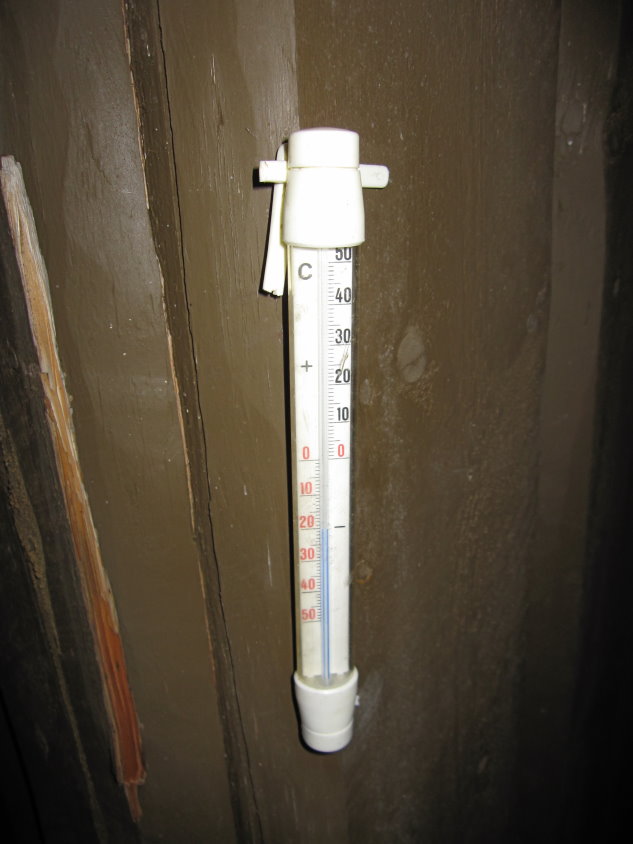This exterior image captures a limited view, revealing the corner of a structure that appears to be either a building or a fence. The wooden surface is coated in brown paint, which is peeling in several areas to expose the underlying wood. Affixed to this corner is a cylindrical thermometer designed to measure temperatures in Celsius. The thermometer features a white cap on both ends and displays temperatures ranging from -50°C to 50°C. The negative temperatures on the left side are marked in red, while the positive temperatures on the right are marked in black. In this shot, the thermometer reads -20°C. Shadows are present at the bottom of the structure, suggesting the image might have been taken in low light conditions, possibly illuminated by an outdoor light or a flashlight.